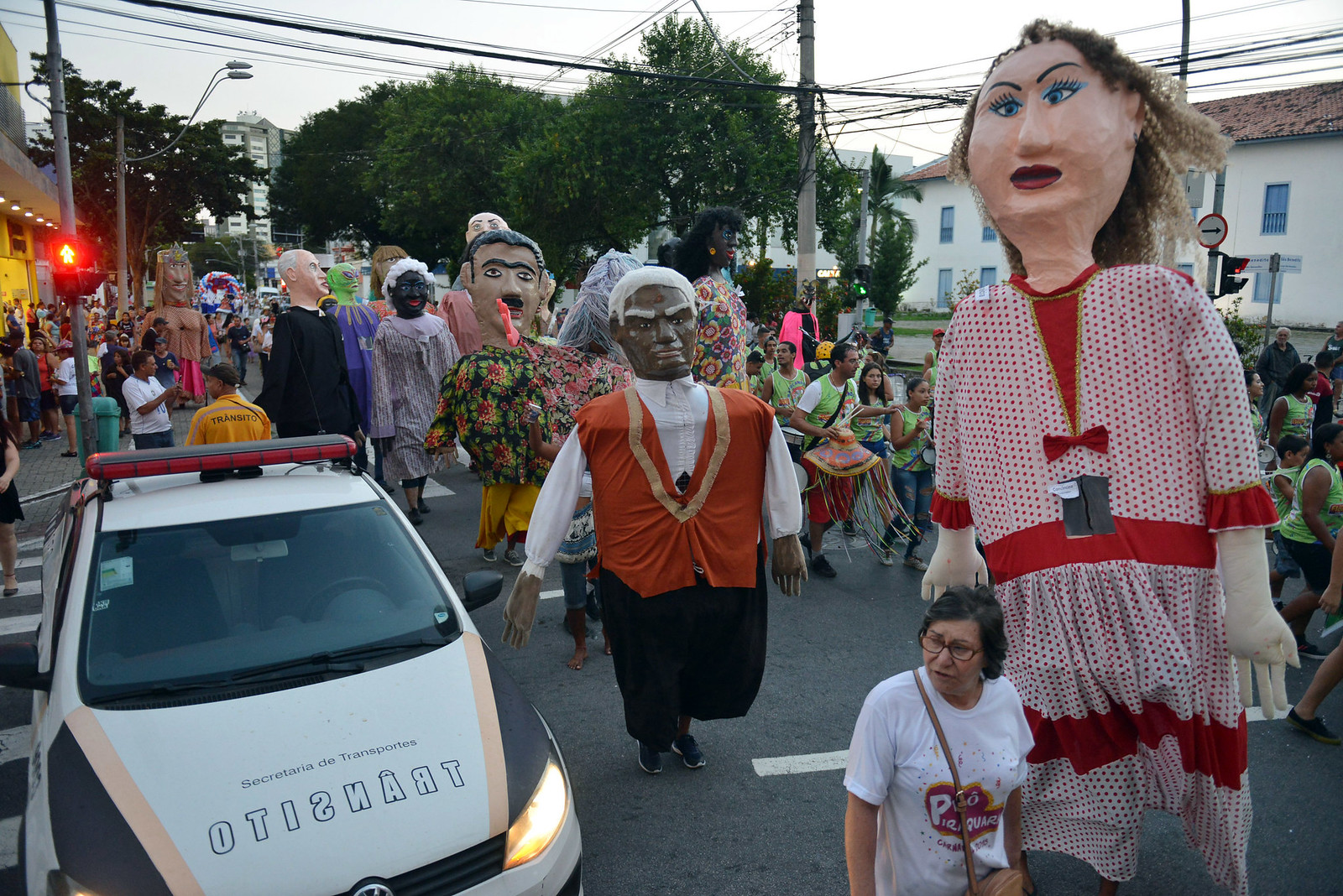The image captures a vibrant outdoor parade scene during the daytime, with various large, human-sized piñatas or mummy-like figures being worn by participants. The piñatas include a striking female figure dressed in a red outfit and a black man adorned in a white and black ensemble with an orange vest. The towering stature of these piñatas is notable, with the heads reaching significant heights above the wearers. The scene is bustling with people walking along the street, surrounded by low buildings, trees, and electric poles. A police car with sirens is parked nearby, adding to the organized atmosphere. In the background, a street sign indicates a crosswalk with a red signal, advising pedestrians not to walk. This lively event is set against a backdrop of urban greenery and distant buildings, further highlighting the community's festive spirit.